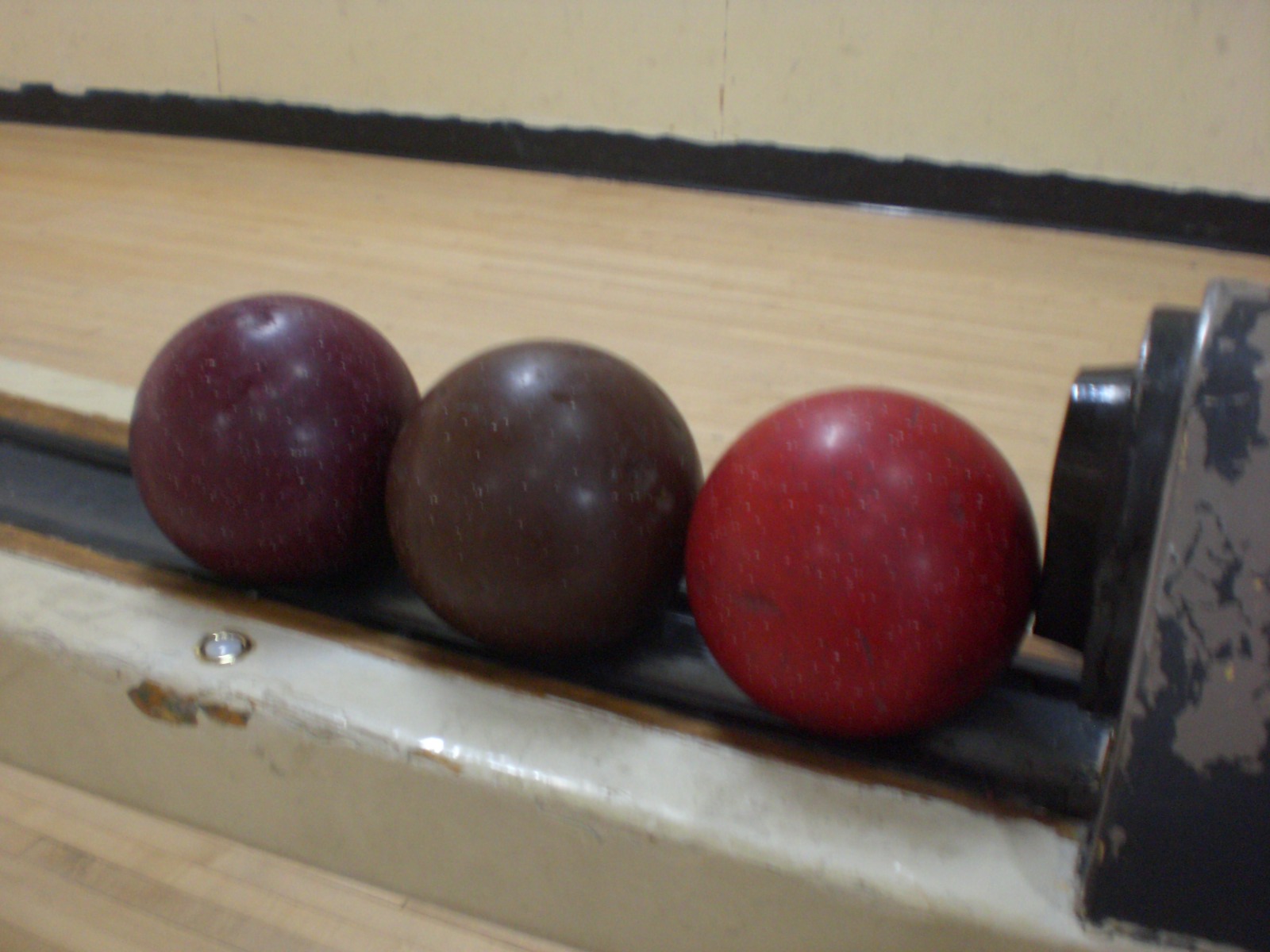This detailed image captures three diverse bowling balls positioned on a return rack. Each ball sports distinct colors and patterns: the leftmost ball is a deep burgundy maroon with light white speckles, the middle ball is a dark chocolate brown with similar speckles, and the rightmost ball is a bright cherry red featuring white speckles and faint gray streaks. The balls are arranged diagonally, with the right one being closest to the viewer and the left one being farthest, all aligned on a black tray that spans most of the image horizontally.

The ball return system, situated beneath the balls, has a chipped blue exterior with black trim and a gray conveyor belt center flanked by two brown stripes. The return is housed in a beige metal platform, prominently scratched and worn, particularly around the edges. To the right, a large, round mechanism with a black center facilitates the release of the balls.

In the background, a light wood-grain bowling lane extends horizontally, bordered by a black edge on one side and the ball return on the other. Above the lane, a white wall with a black border angles slightly downward to the right, completing this intricate and vibrant portrayal of a bowling setting.